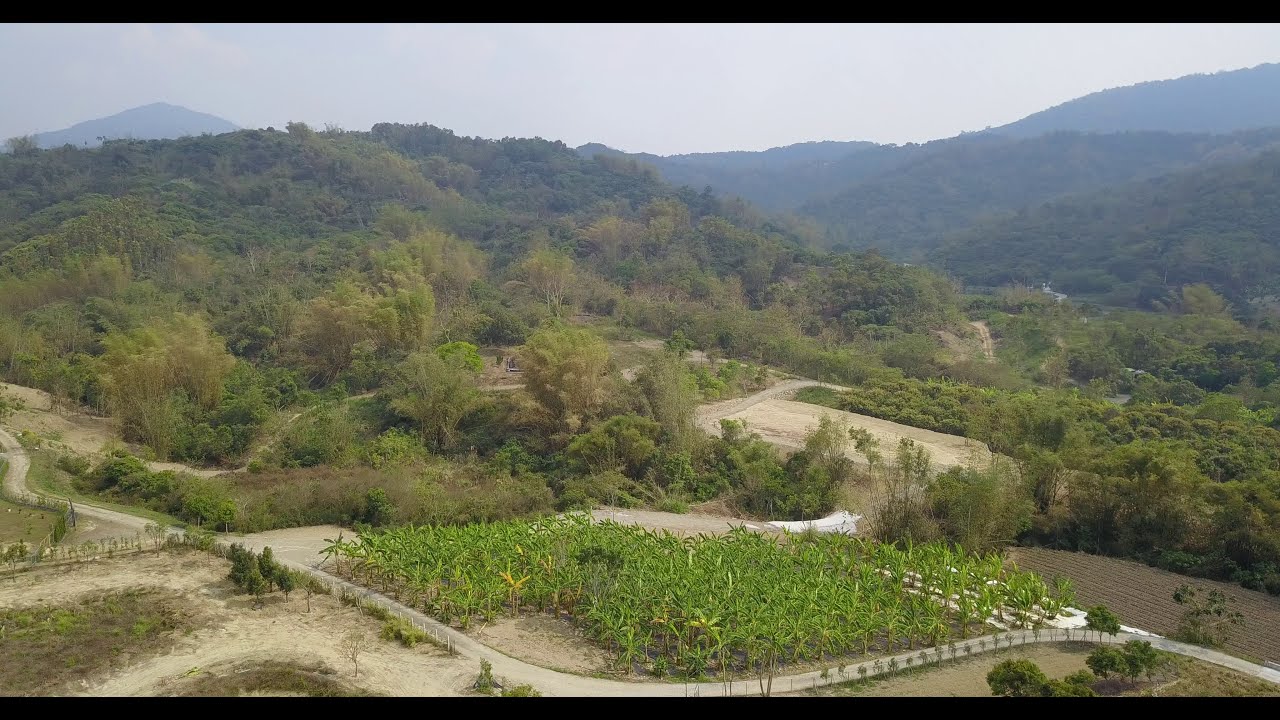This photograph captures a diverse countryside landscape taken during daylight. In the foreground, there is a dirt area leading into a curved road that meanders through the scene, starting from the top left, winding down to the bottom center, and curving outward again towards the top right. Directly adjacent to the road sits a palm tree farm, laid out in zigzag or curved patterns, indicative of deliberate planting. The soil here is light brown and sandy, interspersed with patches of dark brown and green vegetation. Beyond the palm trees lies a field that appears recently planted but not yet fully grown, transitioning into a ditch or small valley lined with additional trees and vegetation. The terrain then ascends into a hill covered in wild vegetation. In the background, the landscape extends into more hills, covered in a mixture of trees and shrubbery, with distant mountains faintly visible through a hazy, partially overcast sky. This combination of cultivated farmland and rugged, natural terrain creates a harmonious blend typical of the countryside.